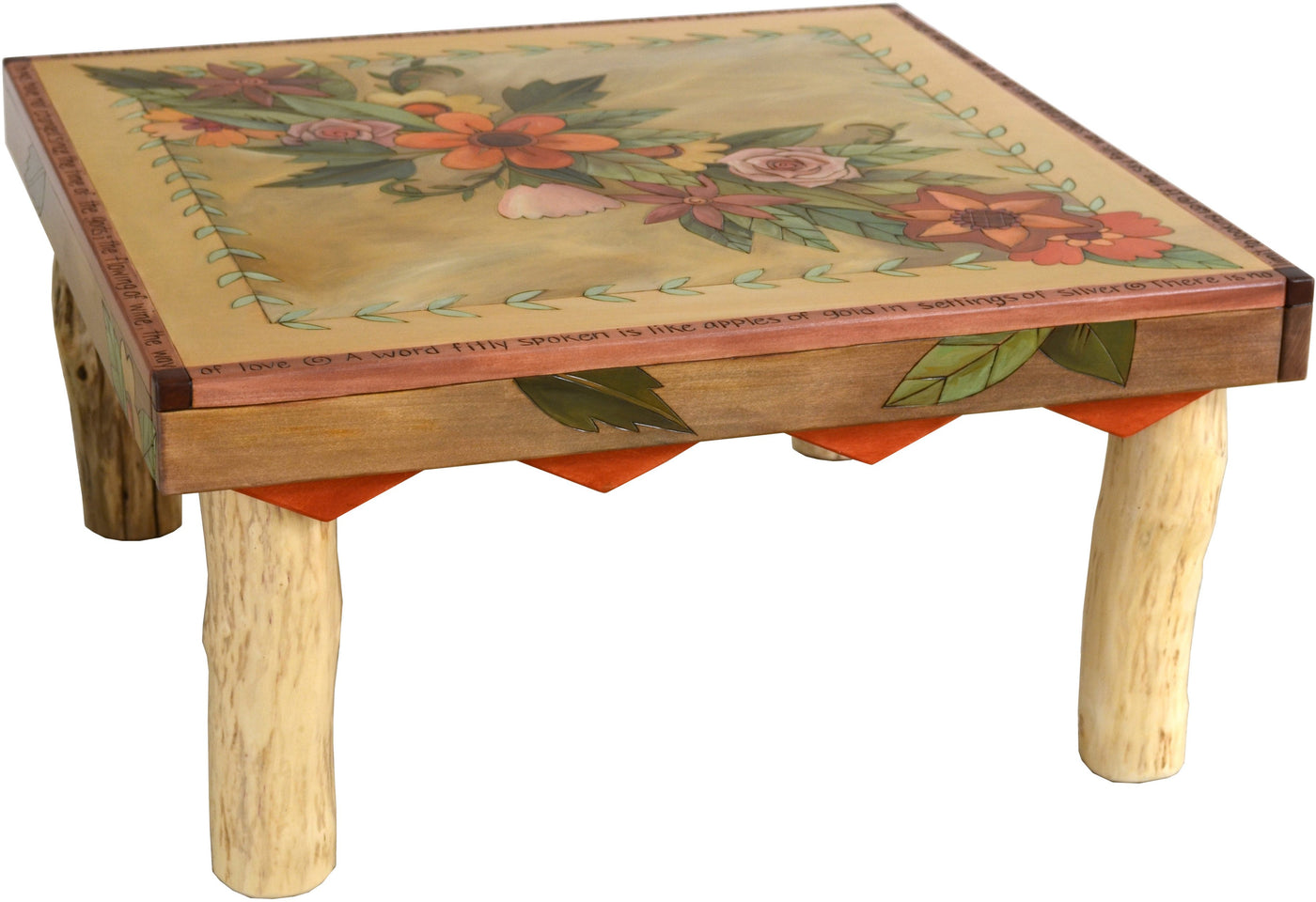This image features a square wooden table with no background, emphasizing the table itself. The legs resemble small, sanded-down tree trunks, giving it a rustic, stool-like appearance. The table is bordered by intricate carvings that seem to contain sentences, although most of the text is unreadable except for a partial phrase: "something spoken is like apples of gold in settings of something." Within the main square, there is a couple inches of plain brown wood followed by a black-outlined square adorned with green leaves along its border. Dominating the center of this inner square is a large orange flower, extending diagonally from one corner to the opposite corner. Accompanying this standout floral centerpiece are several other flowers, including pink roses, a brownish-reddish flower, a red and yellow flower, all interwoven with leafy vines.